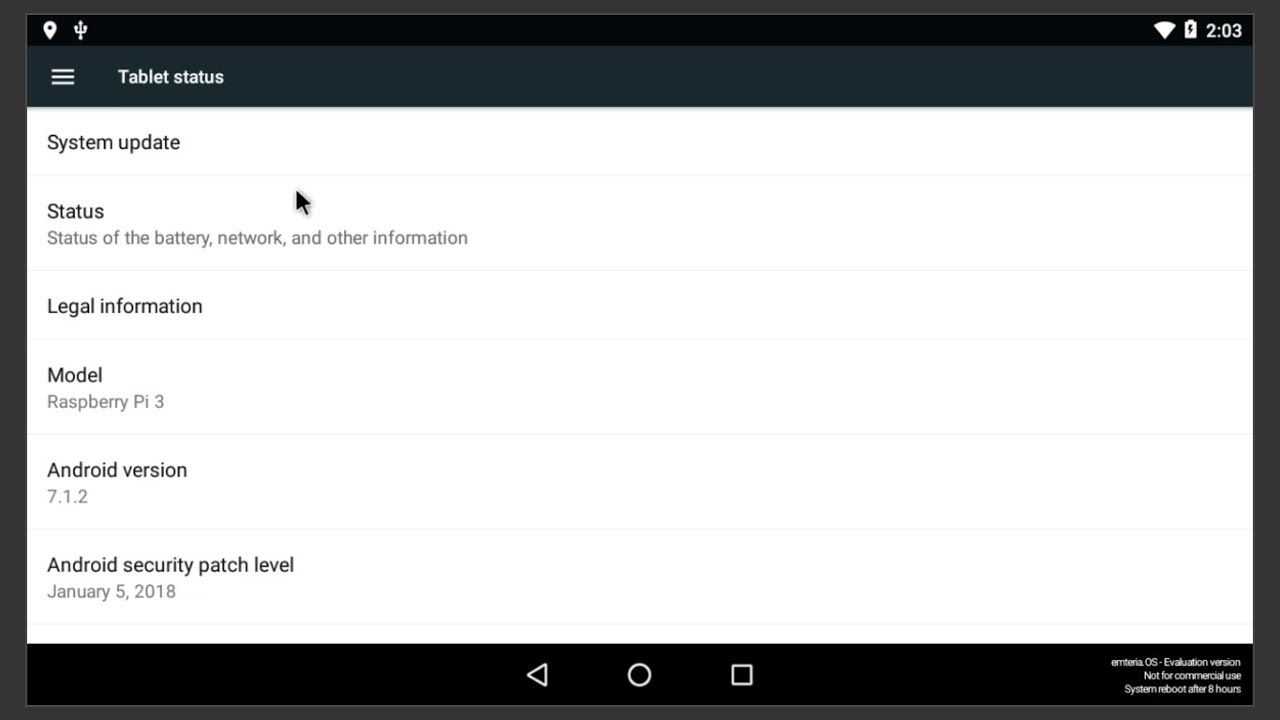The image is a detailed screenshot of a tablet's system information and settings section. The top portion of the image features a dark gray, almost black bar typical of Android or iPhone devices in a panoramic format. From left to right, the bar includes a white location icon and a white symbol resembling a trident. On the far right of the bar are a white Wi-Fi icon, a white battery symbol with a black lightning bolt, and the time displayed as 2:03.

Beneath this, there is a darker gray bar with the left side displaying three stacked white bars, and next to it, the text "Tablet Status" in white. The main section of the image is a large white area divided by thin, faint gray lines, segmenting various pieces of information. At the top in bold black text is "System Update." Below this, labeled "Status" in black, with grey text describing it as "Status of the battery, network, and other information." Further down, there is "Legal Information" in black, followed by "Model," with the inner text indicating "Raspberry Pi 3."

Continuing down the list, it states "Android Version" with "7.1.2" in the corresponding field. Below this is "Android Security Patch Level" noted as "January 5, 2018." Finally, towards the bottom of the image, there is a long black bar featuring a central play button represented by a white triangle in a black-centered white-rimmed circle. To the right are additional control icons, also depicted as white-rimmed circles with black interiors. In the lower right corner of the image, three rows of fine white text can be seen, though they are too small and blurry to be legible. The middle row seems to suggest "not for commercial use," and the last might be "system reboot after eight hours," while the top row appears to be an impractical directive.